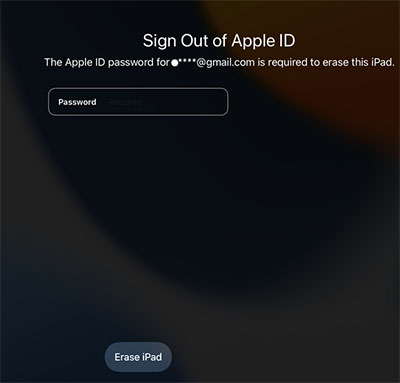The image displays a square screenshot of the Apple sign-out page. At the top, there's a centered header that reads, "Sign out of Apple ID." Below this, text reads, "The Apple password for dot, dot, dot, dot@gmail.com is required to erase this iPad." This line of text is almost flush to the right side of the image. Beneath it is a rectangular password field with curved corners and the word "Password" inscribed inside. At the bottom of the image, a gray capsule-shaped button with white text saying "Erase iPad" is positioned, inset about one-third of the way from the left. The background is a swirling blur with hues of purple, hints of orange, and lighter gray tones concentrated in the upper right and lower left corners. Overall, the alignment of elements seems inconsistent and visually unbalanced, which is uncharacteristic of Apple's typically precise design standards.